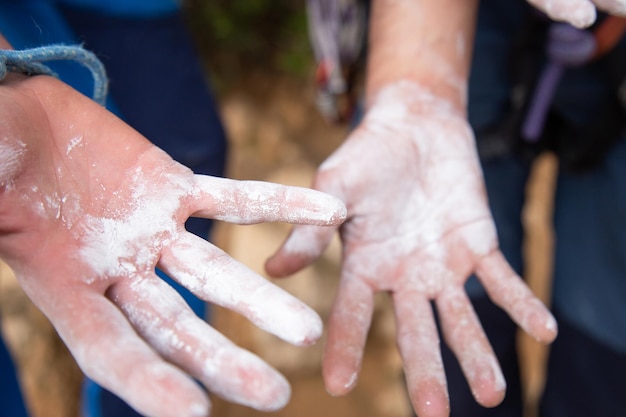In this photorealistic image, captured from a top-down perspective, the focus is on the right hands of two young individuals extending their palms towards the camera, covered in a fine white powder, likely chalk. The background is intentionally blurred, with hints of green and brown, suggesting an outdoor, natural setting. Both individuals are dressed in dark blue clothing and wear ropes around their waists and the left wrist, indicating they might be rock climbers. The left hand, partly covered in chalk, has streaks across the palm and full coverage on the fingers, while the right hand is almost entirely coated, with some spots on the fingertips missing. The overall visual emphasizes the texture of the chalk and the youthfulness of the hands, providing a striking contrast against the blurred backdrop.